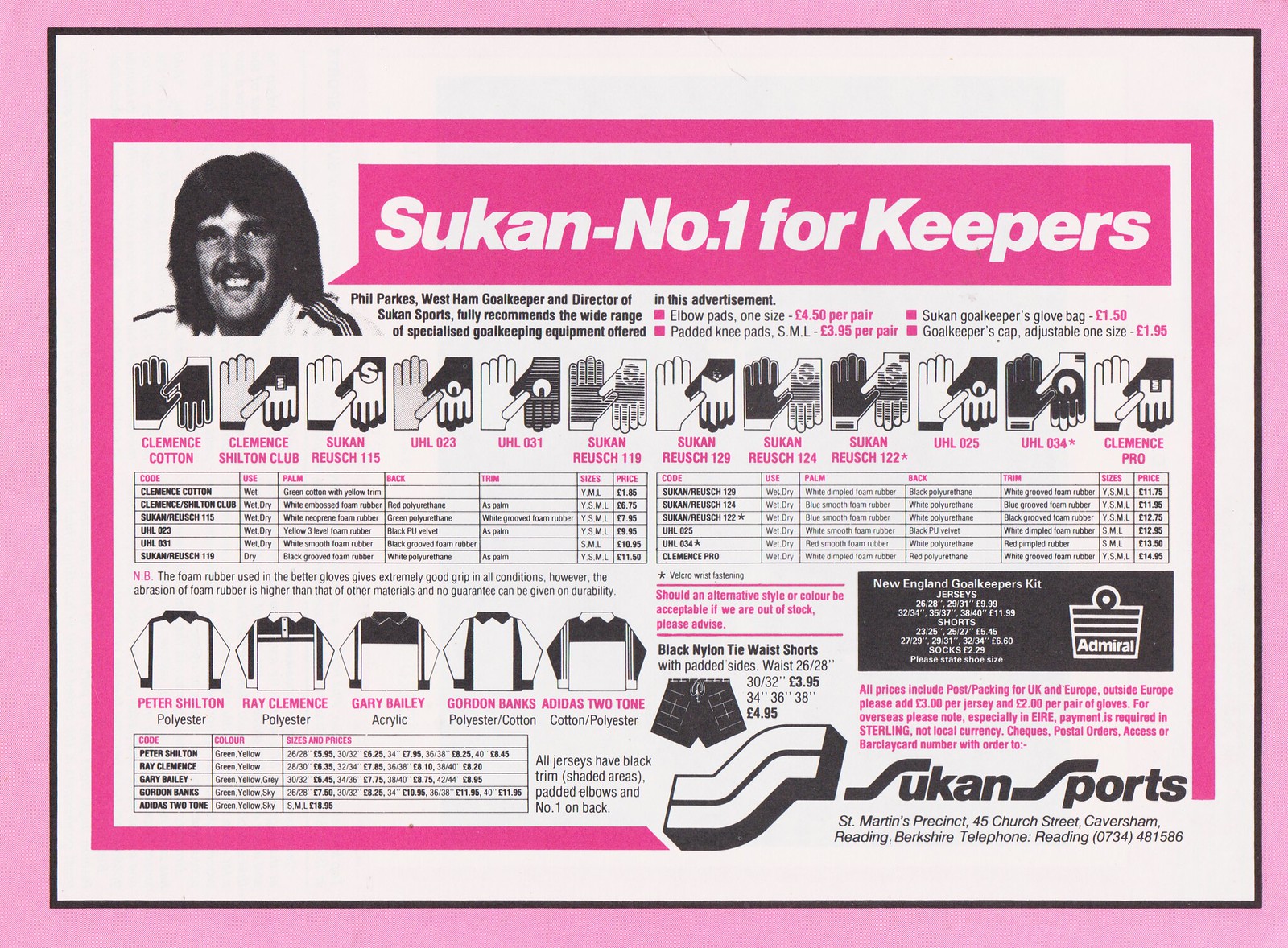A detailed caption of the image would be:

This is a scanned page, likely from an old magazine or possibly an old advertisement. It features a double pink border, with a white border sandwiched in between, and a central white section. Dominating the top is a black-and-white photo of a smiling man with long dark hair and a mustache, wearing a white shirt with black stripes on the sleeves. Encasing his headshot is a pink speech bubble with white text that reads, "Sukan - Number One for Keepers." Beneath, in black text, it states, "Phil Parkes, West Ham goalkeeper and director of Sukan Sports, fully recommends the wide range of specialized goalkeeping equipment offered in this advertisement."

The page showcases numerous detailed, sketched images of different types of goalkeeping gloves with names such as Clemens Cotton, Clemens Shelton Club, Rukan Rush 115, UHL 023, UHL 031, Sukan Rush 119, Sukan Rush 129, Sukan Rush 124, Sukan Rush 122 asterisk, UHL 025, UHL 034 asterisk, and Clemens Probe. Each glove image is accompanied by extensive specifications including sizes and materials.

Lower on the page, there are illustrations of various goalkeeping shirts: Peter Shelton (polyester), Ray Clemens (polyester), Gary Bailey (acrylic), Gordon Banks (polyester/cotton blend), and Adidas two-tone cotton/polyester. Additionally, there are images of elbow pads, padded knee pads, a goalkeeper’s glove bag, and an adjustable goalkeeper’s cap. At the bottom, there is an illustration of black nylon, tie-waist shorts with padded sides.

The advertisement lists the shop's details: Sukan Sports located in St. Martins Precinct, 45 Church Street, Caversham, Reading, Berkshire. It also includes a telephone number for orders or inquiries: Reading 0734-481586.